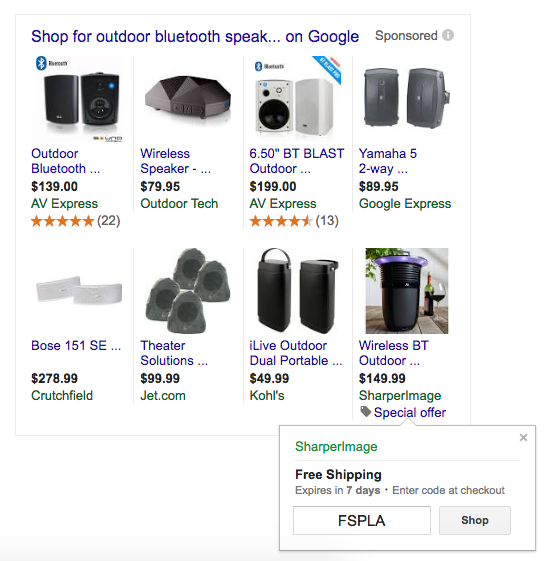Explore the best outdoor Bluetooth speakers available on various platforms:

1. **AV Express Wireless Speaker**: Priced at $79.95, this versatile speaker offers robust audio quality for all your outdoor activities.
2. **Outdoor Tech 6.5 Inch BT Blast**: Available for $199 at AV Express, this speaker boasts powerful sound and Bluetooth connectivity, perfect for any adventure.
3. **Yamaha 5 Two-Way Speaker**: Priced at $89.95 on Google Express, this reliable Yamaha model ensures clear and precise audio outdoors.
4. **Bose 151 Speaker**: Available for $278.99 at Crutchfield, this premium Bose speaker delivers exceptional sound quality with durability suited for outdoor use.
5. **Theater Solutions Outdoor Speaker**: Priced at $99.99 on Jet.com, this speaker provides a great balance of performance and value.
6. **I Live Outdoor Dual Portable Speaker**: Available for $49.99 at Kohl's, this portable speaker is ideal for those on the go, offering wireless convenience and great sound.
7. **Kohl's Wireless BT Outdoor Speaker**: Priced at $149.99, this wireless option from Kohl's combines quality and affordability for outdoor entertainment.
8. **Sharper Image Special Offers**: Take advantage of free shipping on wireless Bluetooth outdoor speakers from Sharper Image, available for a limited time with the code "FS PLA" at checkout.

Find the perfect outdoor Bluetooth speaker for your needs and enjoy exceptional sound quality, no matter where you are.